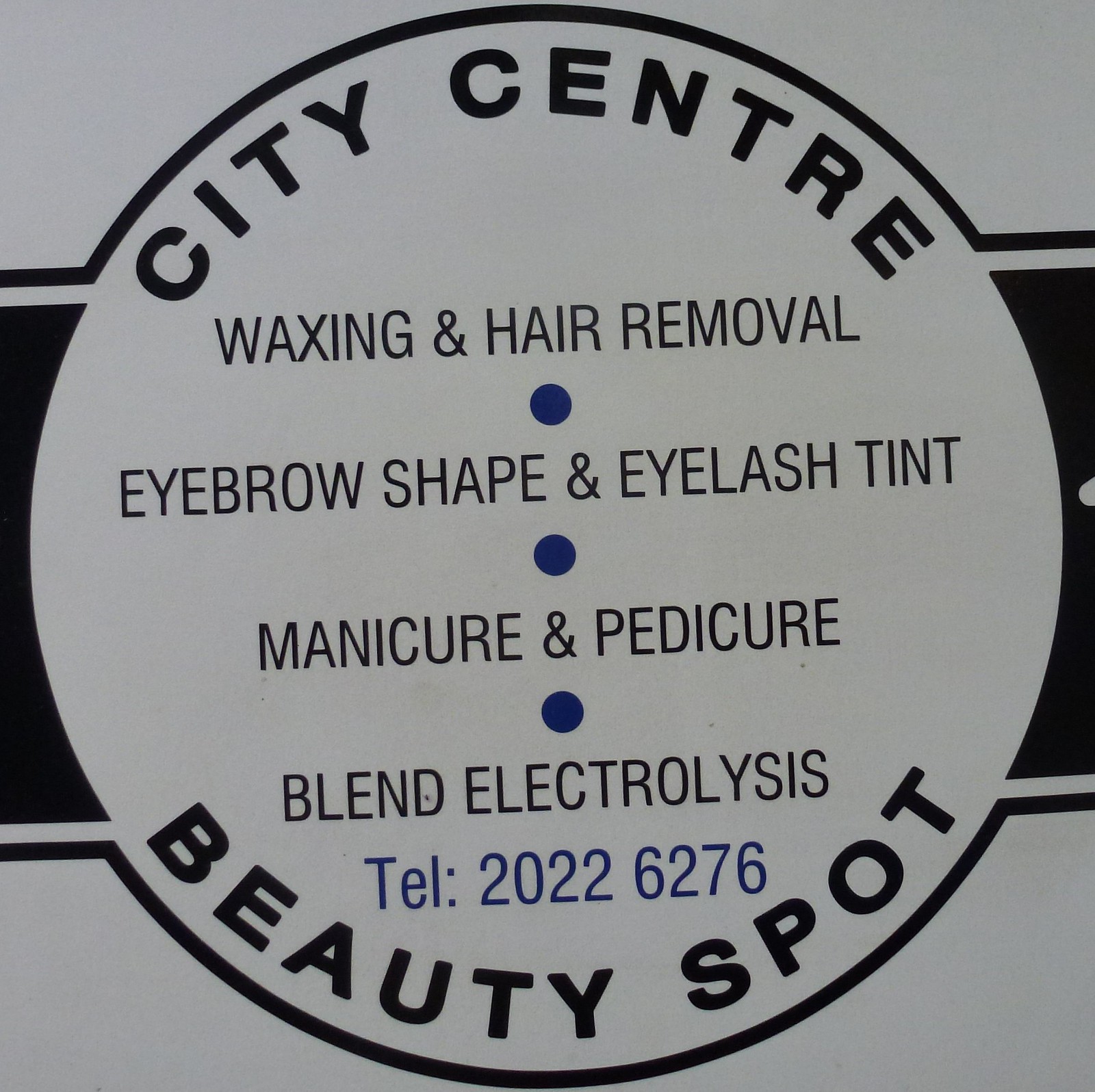The image features a business sign with a light gray background and a prominent circular design. The circle has the words "CITY CENTRE" in bold, black letters arcing along the top. Below this, in centered horizontal text, it lists "WAXING AND HAIR REMOVAL." This is followed by a sequence of services separated by small blue dots: "EYEBROW SHAPE AND EYELASH TINT," "MANICURE AND PEDICURE," and "BLEND ELECTROLYSIS." Towards the bottom, it includes the contact detail in blue letters: "TEL: 2022-6276." Finally, the words "BEAUTY SPOT" are displayed in bold letters, curving along the bottom perimeter of the circle. The sign is likely mounted on a building and has a black stripe or line in the background, enhancing its visibility.